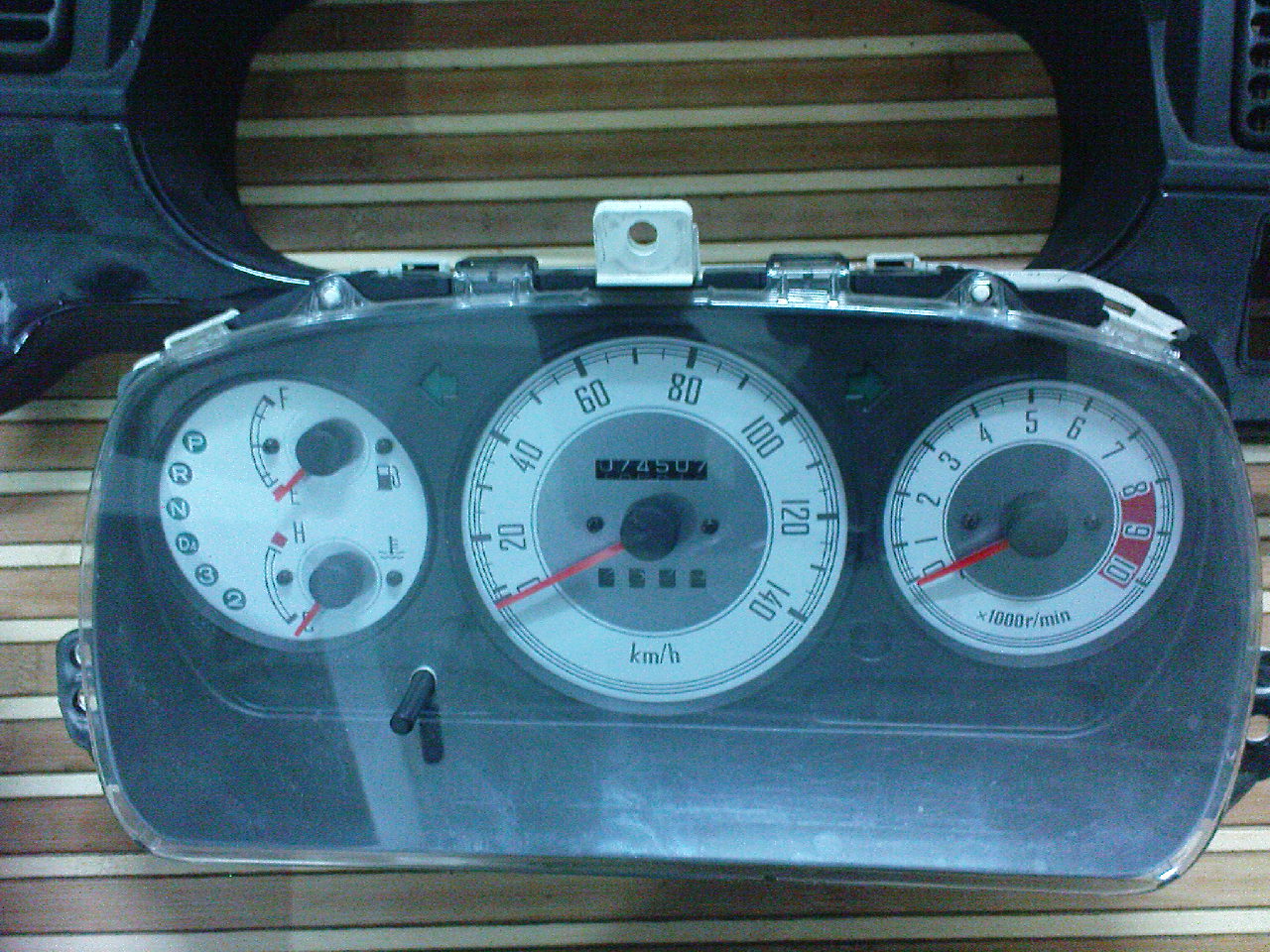This image features a detached car instrument cluster, likely from the dashboard of a vehicle. The device is predominantly black and rectangular with rounded edges, resembling the area typically found behind the steering wheel.

On the left side of the instrument cluster, there is a smaller round gauge. This gauge has a white background, indicating fuel levels with the standard "Full" and "Empty" markers and a small gas pump icon accompanied by an oil temperature reading, displaying "High". Below this is an arrangement of gear indicators listed as "P, R, N, D, 3, 2", aligned along a green curve.

In the middle of the cluster, there is a larger round gauge, clearly marked from 0 to 140 along its top edge, identifying it as the speedometer. The speed is denoted in kilometers per hour (km/h). Flanking this central gauge are two arrows, one pointing left and the other right, signifying turn signal indicators.

On the far right of the cluster is another gauge, similar in size to the leftmost one. This gauge is marked from 0 to 10, where the bottom label reads "10 R/M", which likely refers to revolutions per minute (RPM), an indicator of engine speed.

These features collectively confirm that this piece is indeed an essential component from a car's dashboard, although it has been removed from its original setting.